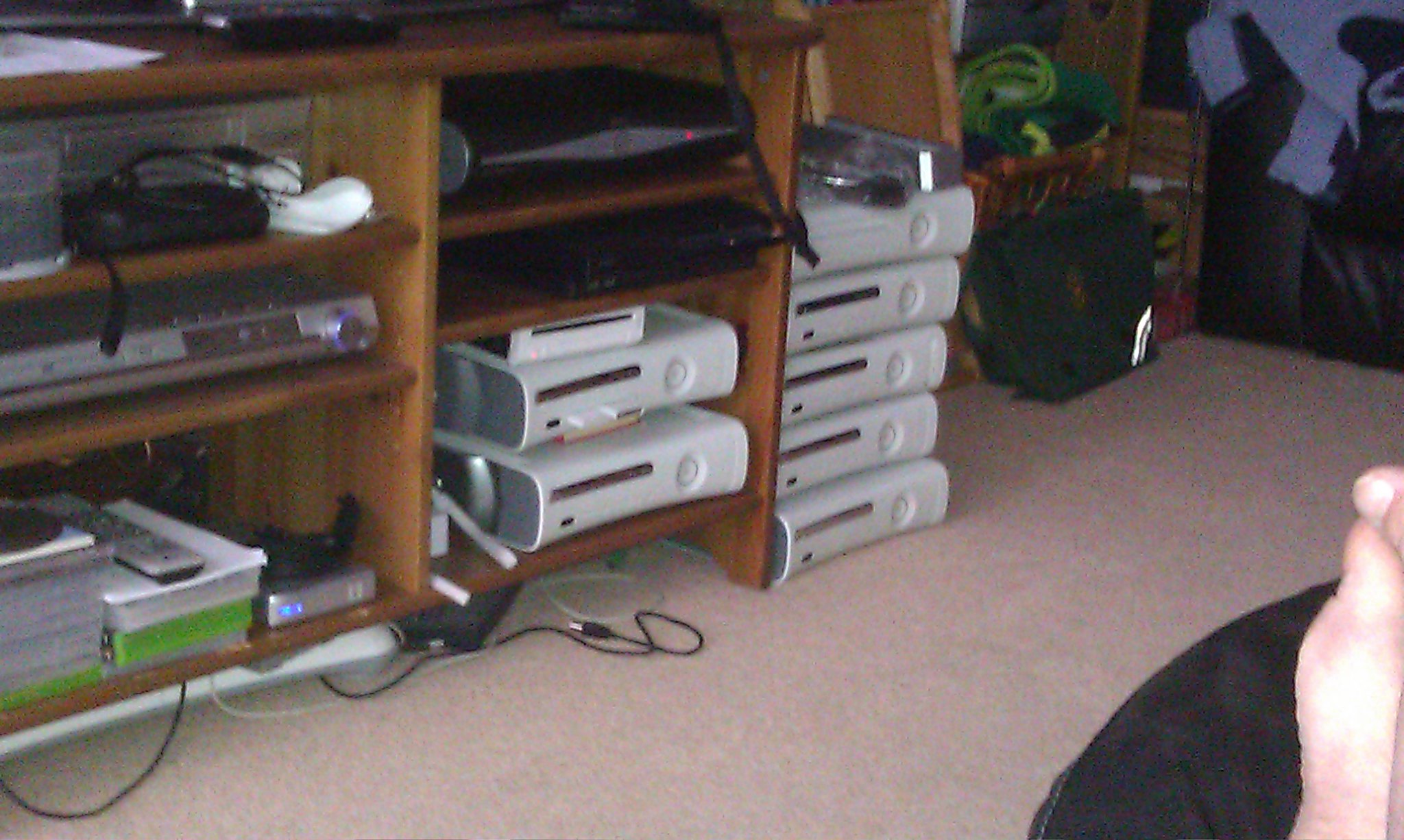The photograph captures a detailed view of a wooden entertainment center laden with electronic devices and video game equipment. On the bottom left shelf, there are multiple green boxes, clearly video game cases, topped with a rectangular white remote control. A digital receiver with a large metal knob and a black LED screen occupies the next shelf above. The shelf above that is home to a white video game controller and a black box with black headphones resting on it. Situated on the bottom right of the entertainment center, two white Xbox consoles are stacked on top of each other. Adjacent to this stack, on the floor leaning against the right side of the entertainment center, is an additional stack of five Xbox consoles. The very bottom right of the image reveals the bare feet of an individual resting on a beanbag, adding a casual touch to the scene. Off to the side, partly visible, there might be what appears to be a thin metal DVD player and possibly a PlayStation 2, contributing to the array of electronic devices.